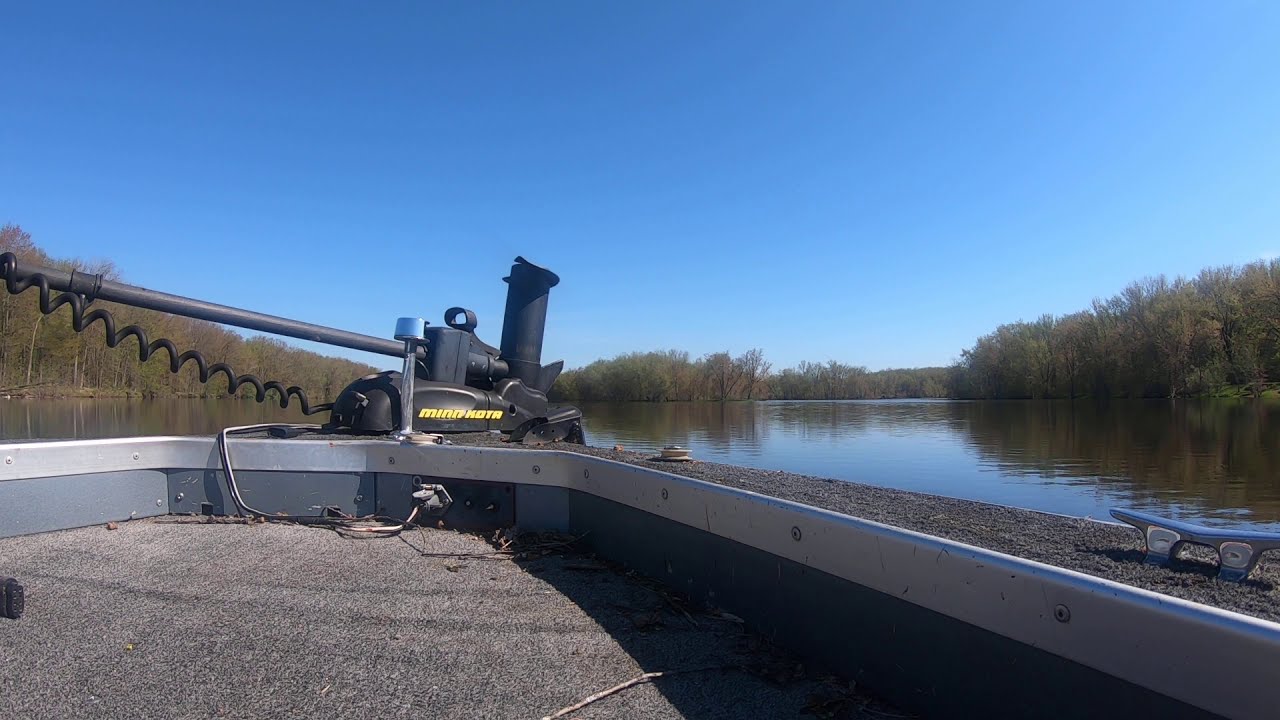A daylight photograph captures the scenic view from within a boat, likely a skiff, on a body of water that could be a river, pond, or lake. The bottom and left side of the image are dominated by the boat's interior, featuring a textured black deck designed to prevent slipping when wet, bordered by silver railings. A prominent black trolling motor with a coiled wire extending from it is situated near the front or possibly the aft end of the boat. This motor features a yellow label reading "MINKOTA." The water surfaces are calm with some light ripples and reflect the clear, light blue sky and dense green foliage of the shoreline trees. Trees line both sides of the waterway, extending from nearby to the distant background, creating a natural, tranquil setting. The setting is vividly illuminated by daylight, suggesting it was taken during the daytime.